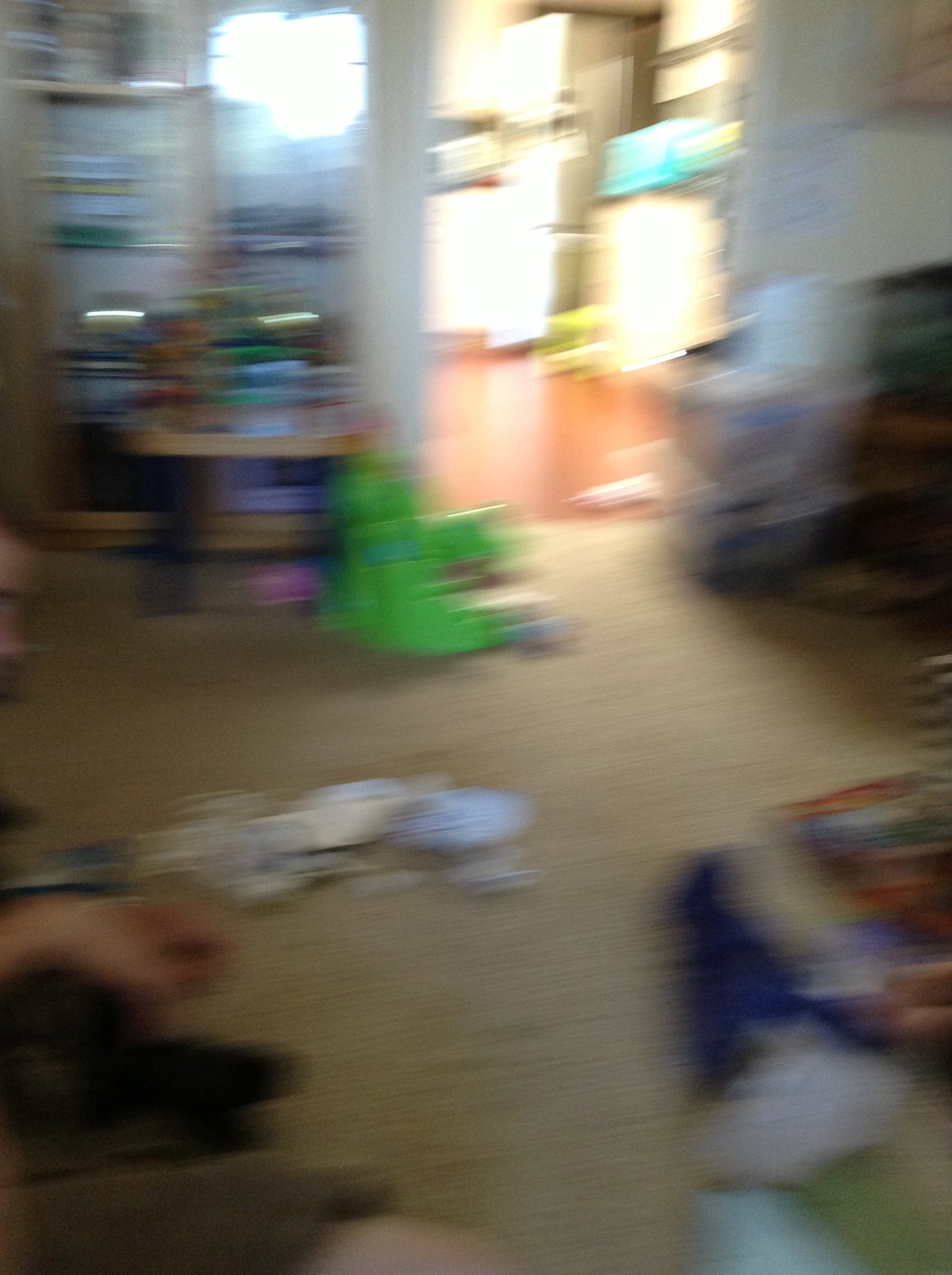In this blurry photograph taken inside a house, the primary focus seems to be on various children's toys scattered across the floor. Among them, there appears to be a large, green object, possibly a dinosaur toy, though it's difficult to confirm due to the image's lack of sharpness. The scene is set in what looks like the living room, extending towards a more brightly lit kitchen area in the background. The lighting contrast makes the kitchen more visible, while the living room remains dim. On the left side of the frame, part of someone's hand is faintly visible, indicating that the camera was in motion when the picture was taken. Interestingly, despite the blurriness, some trees outside the house are distinctly visible through a window.